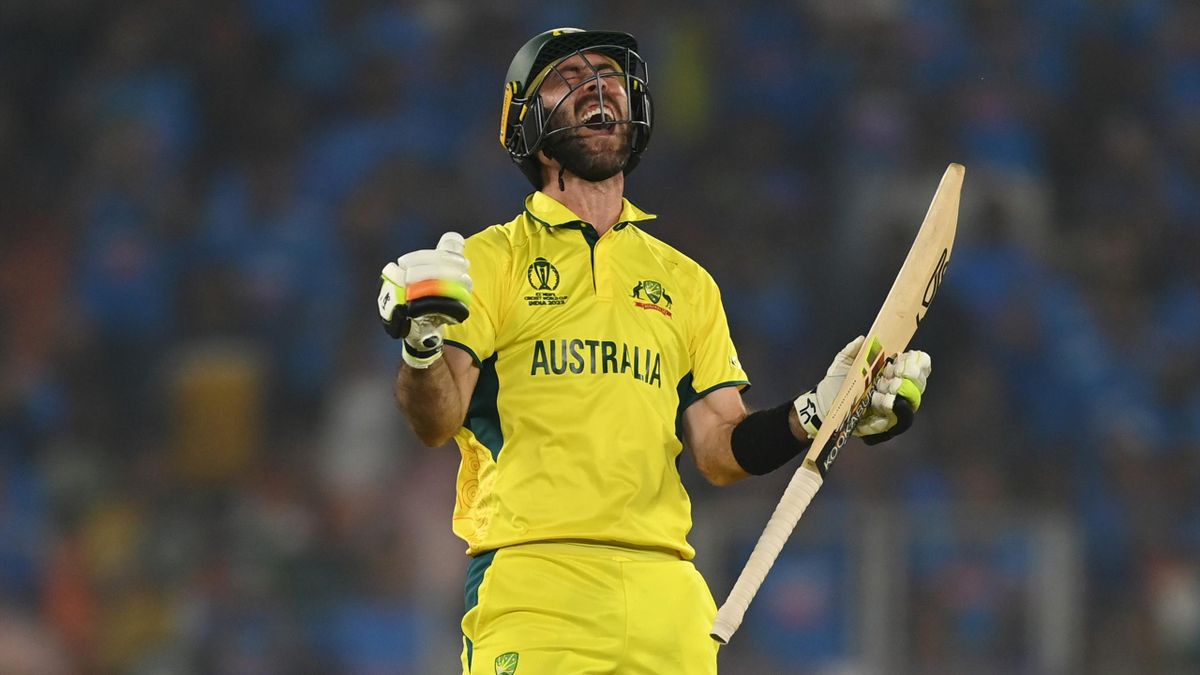The image depicts a jubilant sports player, apparently a cricket player, positioned centrally against a blurred backdrop of a crowd. The man, facing the camera, is dressed in a yellow collared polo shirt, which prominently features the word "Australia" written across the front in dark letters. Accents of black or possibly dark green trim are visible around the zipper, buttons, and just under his armpits. He dons matching yellow shorts with a black stripe down the side at the hip. His attire is complemented by white gloves with intricate details: yellow on the ring fingers, black on the pinkies, and a black band on his left wrist.

The player is in a celebratory pose, with his head tilted back slightly and to the right, mouth open wide in a jubilant scream, and eyes closed, capturing a moment of sheer joy or triumph. He is also sporting a prominent beard and wears a black helmet with a wire face mask. In his left hand, he holds a wooden cricket bat covered in markings. His arms are bent at the elbows, reaching forward, accentuating his exuberant expression.